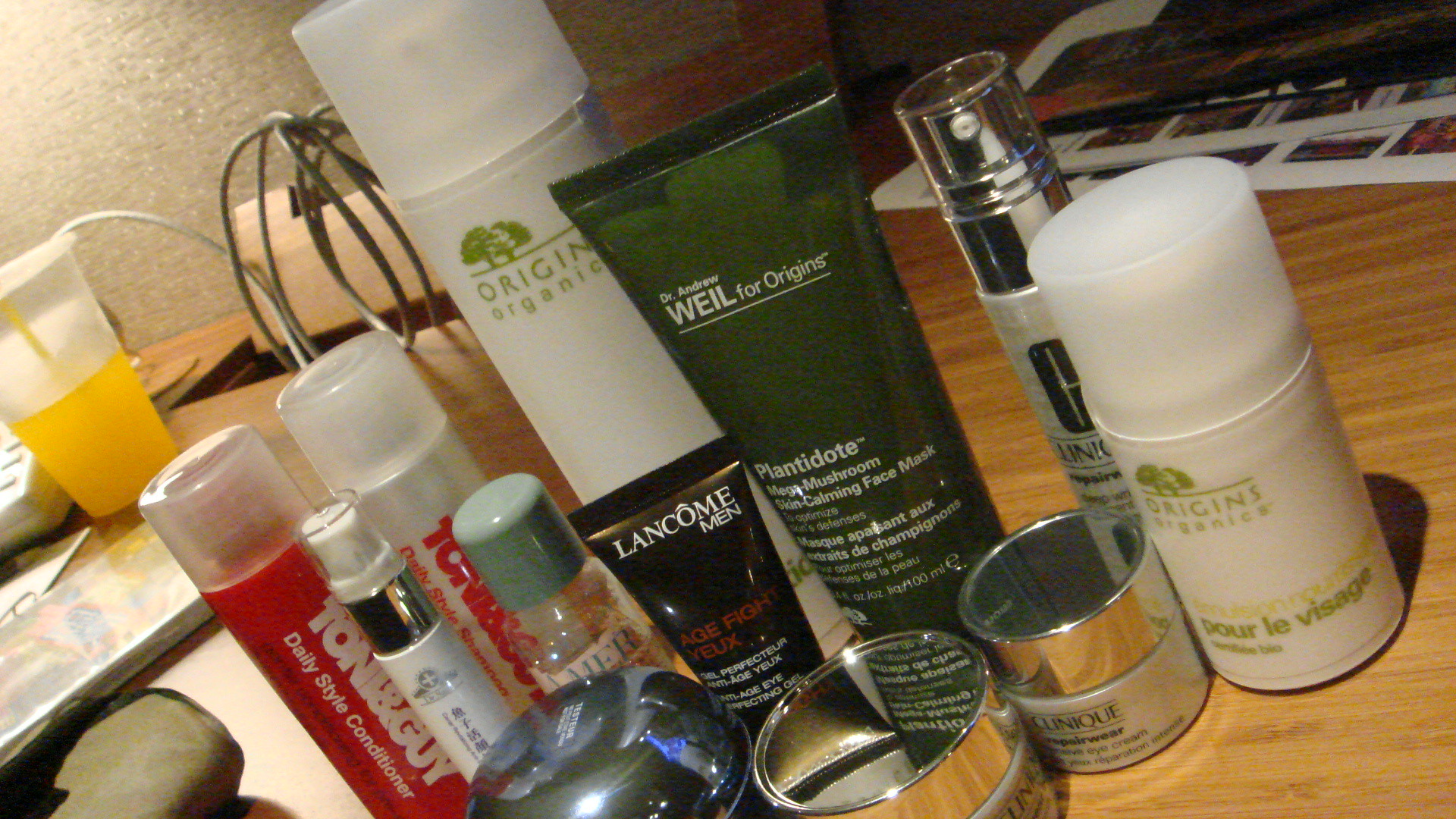Close-up of a Skewed Collection of Men's Skincare and General Care Products

In an angled, close-up shot of a desk, predominantly men's skincare and general care products are displayed in a slightly skewed manner. On the left, a red container with a clear lid labeled "Tony and Guy Daily Style Conditioner" stands out. Nearby, there are smaller containers whose labels are not fully visible—one with an aqua green lid, and a long white container with a clear top.

Towards the front, an all-black bottle shaped like a lotion container reads "One Comb Men" and "Age Fight," with some text in French. Beside it, a large bottle, roughly the size of a hairspray can, has the word "Organic" (or possibly "Generic") on it. 

To the right of this are several products: a blue, lotion-shaped bottle labeled "Dr. Andrew Weill for Origins," a clear spray bottle with a silver cap, and a smaller "Origins" container. In the far-left background, a half-filled cup of orange liquid with a straw is visible. The collection is set atop a desk, accompanied by a wound cable at the back and some papers or photographs on the upper right-hand side.